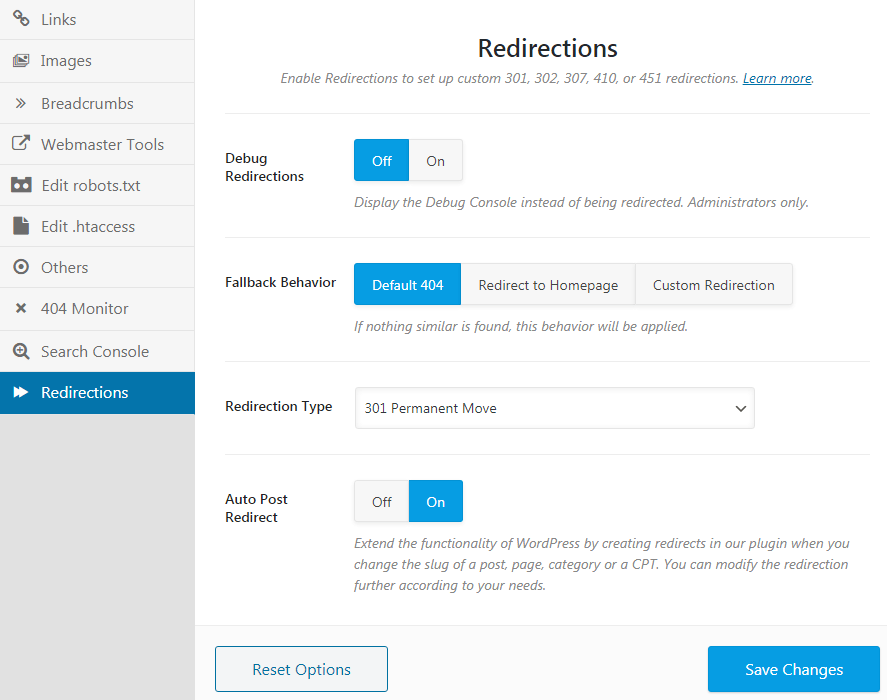The image is a screenshot from what appears to be a web application interface, likely geared towards web development or SEO management. The layout consists of a two-column design. On the left side, there is a vertical navigation menu enclosed within a light gray sidebar. This sidebar contains options labeled as: 

- Links
- Images
- Breadcrumbs
- Webmaster Tools
- Edit robots.txt
- Edit .htaccess
- Others
- 404 Monitor
- Search Console
- Redirections

Notably, the "Redirections" option is highlighted in a blue text box, indicating it has been selected.

On the right side, taking up the majority of the page, is a white background area displaying detailed functionalities related to "Redirections." At the top of this section, the word "Redirections" is prominently displayed. Below this, there are several interactive elements including buttons and drop-down menus. 

- There is a button labeled "Debug Redirections" which appears to be toggled off.
- Another section, "Fallback Behavior," is set to a "Default 404" status.
- A drop-down menu allows for the selection of "Redirection Type."
- There is an option called "Autopost Redirect."

At the bottom of this right-side section, two key buttons are present:

- "Reset"
- "Save Changes"

The overall design employs a minimalist aesthetic with a white background and text in shades of gray and black, ensuring that the interface remains clean and focused on usability.